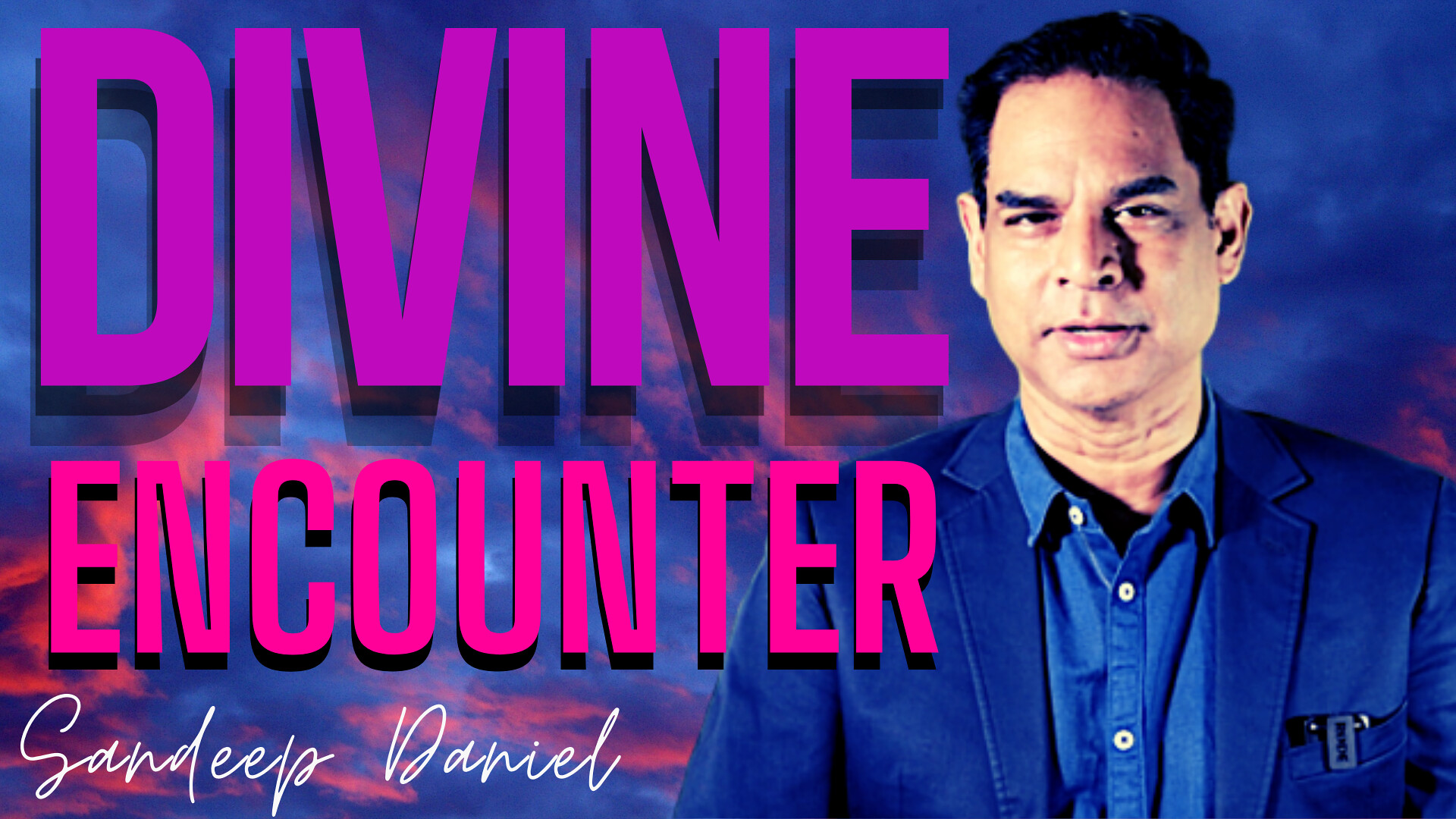The image appears to be an advertisement featuring a man on the right side. The background captures a serene sky transitioning with shades of blue and pink, portraying either a sunrise or sunset with clouds tinged in pinkish-orange hues. Dominating the left side of the image, the word "DIVINE" is prominently displayed in large, purplish letters with a shadow effect, creating a 3D appearance. Below it, the text "ENCOUNTER" is emblazoned in bold hot pink letters. Just beneath these, the name "SANDEEP DANIEL" is elegantly inscribed in white cursive script. The man, presumably Sandeep Daniel, has short wavy black hair, a serious expression, and thick black eyebrows. He’s dressed in a dark blue jacket over a denim button-up blue shirt, possibly featuring a pocket protector. He gazes directly at the camera, adding a personal touch to the promotional image.